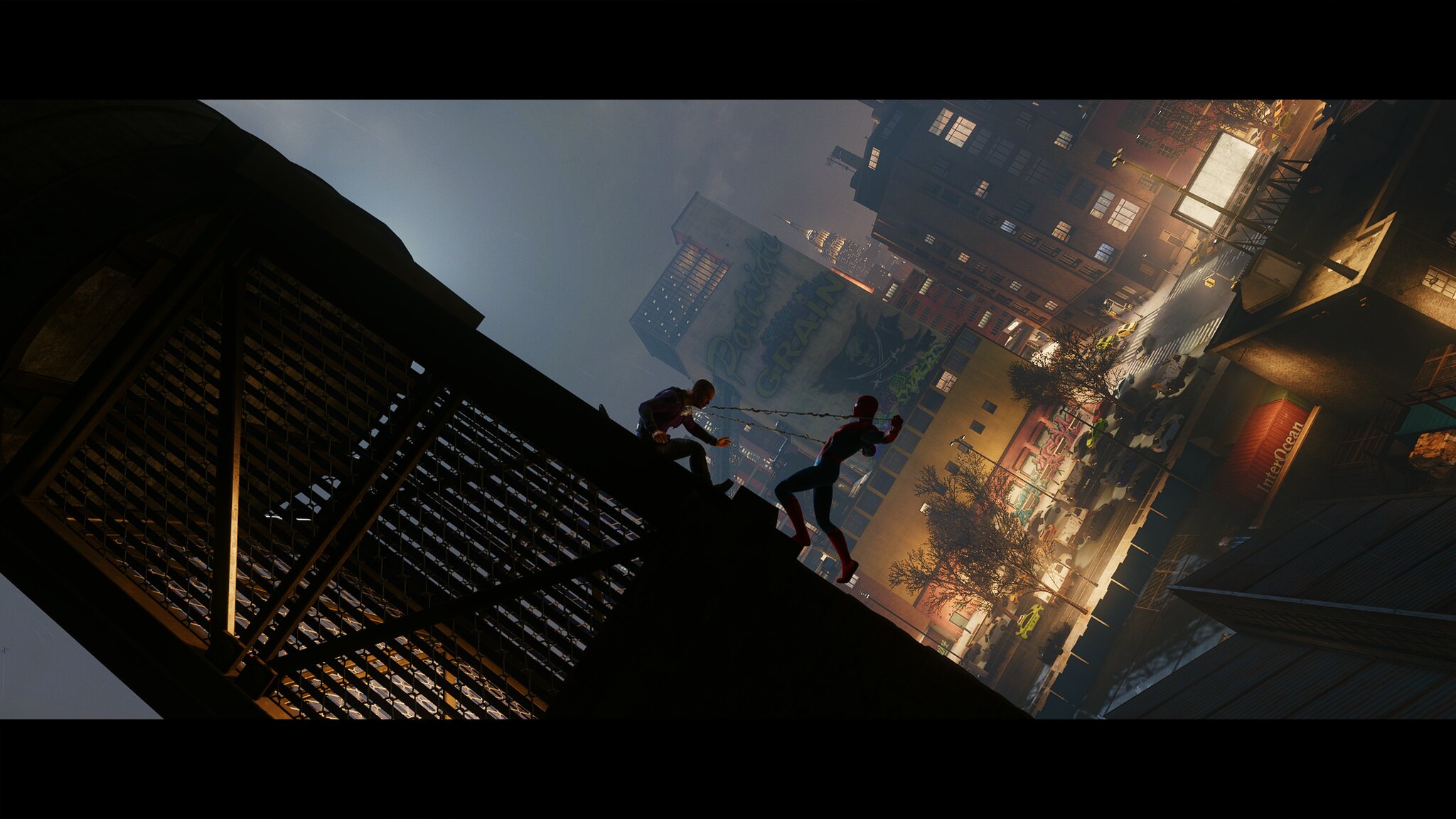In this vividly detailed color image, which seems to be a screenshot from either a film or a video game, two figures are positioned atop a decorative metal structure that resembles scaffolding. The scene is set against the backdrop of a cityscape bathed in the dim, gray haze of night or dusk. In the distance behind them, illuminated buildings and a small parking area with trees are visible, contributing to the atmospheric urban setting.

The figure on the right stands upright with his arms dramatically pulled back, giving the appearance of being ready for action or confrontation. He is dressed in a superhero-like costume, which adds to the dramatic tension of the scene. Opposite him, a second male figure is seated, directly engaged with the standing figure. Their postures and proximity suggest a conflict or intense interaction, rich with narrative implication.

The structure they are on is partially open, allowing some light to filter through and casting a mysterious glow over the scene. The intricate details of the metal structure, combined with the ambient city lights, create a visually striking and tense environment for this pivotal moment.